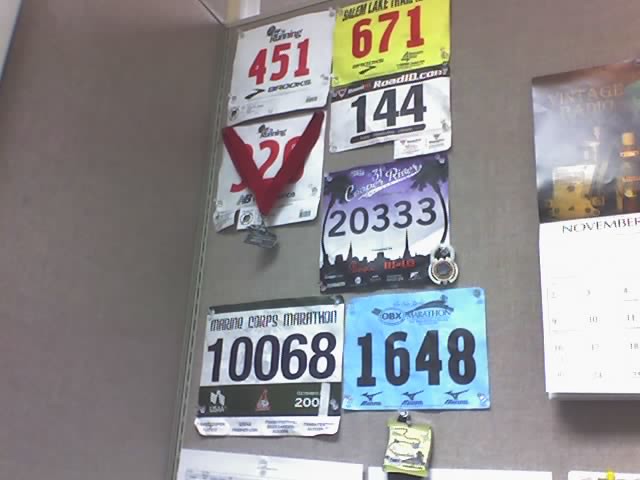The photograph showcases a gray cubicle wall adorned with various marathon race bibs pinned to its surface. Among the noticeable bibs are one from the Marine Corps Marathon displaying the number 10068, and another from the OBX Marathon featuring the number 1648. Additional race tags include one with the number 20333, another with the number 671 from the Salem Lake race, and tags numbered 326, 144, and 451, though some details of these are not entirely legible. All the bibs are arranged neatly, reflecting a sense of accomplishment and a passion for running. To the right of these bibs, a calendar flipped to November is also pinned to the wall, adding a functional element to the display. The gray color of the cubicle provides a neutral backdrop that highlights the various colorful race tags and the calendar.